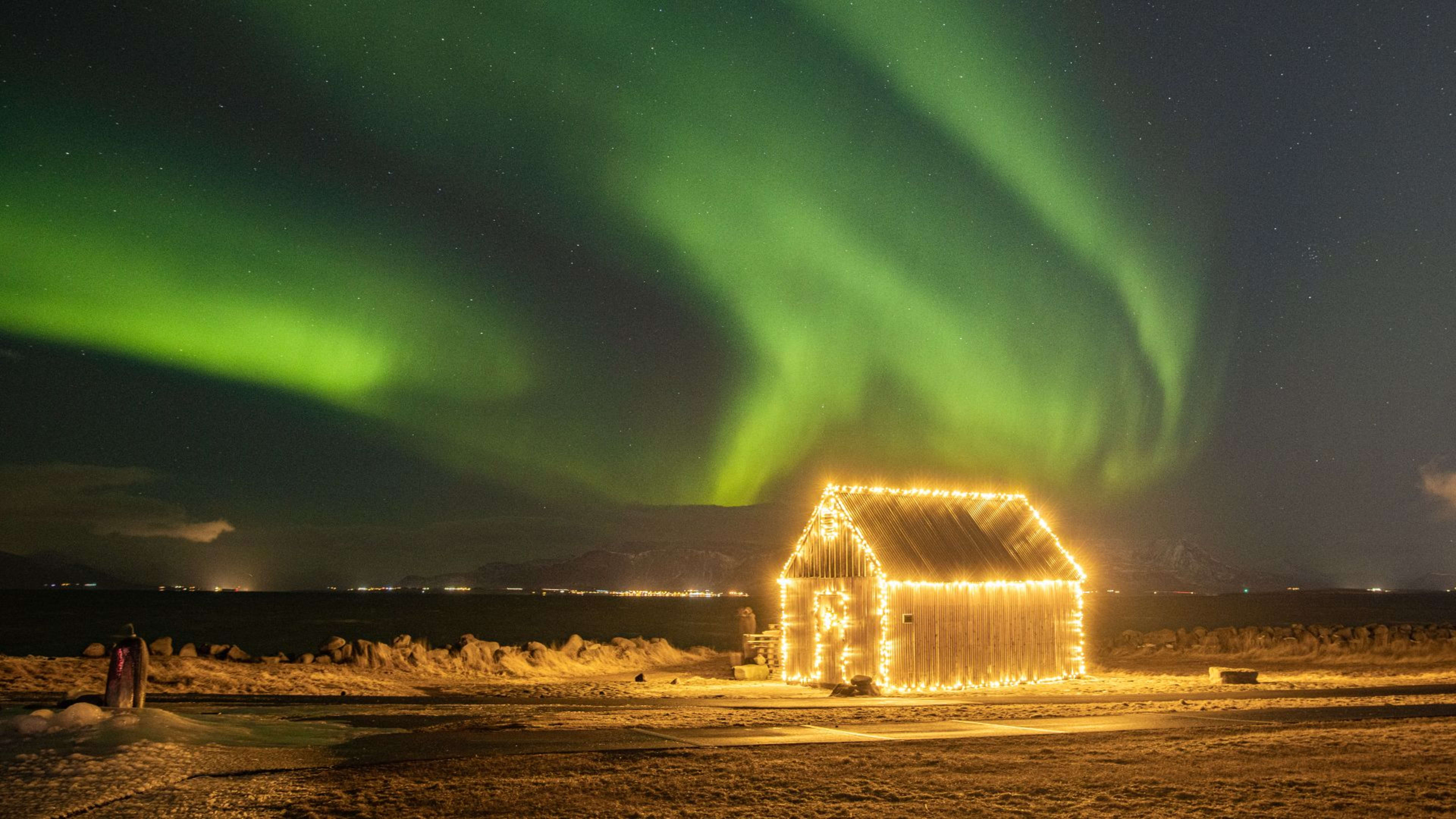This mesmerizing nighttime photograph captures the Northern Lights, or Aurora Borealis, painting the sky in vivid green bands that swirl elegantly amidst a backdrop of twinkling stars. In the foreground, a desert-like terrain stretches out, where a man and a woman stand diminutively in the lower left, gazing in awe at the celestial phenomenon. Dominating the central lower portion of the image is a charming farmhouse-like building, adorned with golden fairy lights that outline its roof and edges, creating a festive glow. Beneath the ethereal lights, distant mountains and sparse clouds add depth to the scene, while a narrow band of city lights subtly illuminates the horizon, enhancing the breathtaking expanse of this natural wonder.